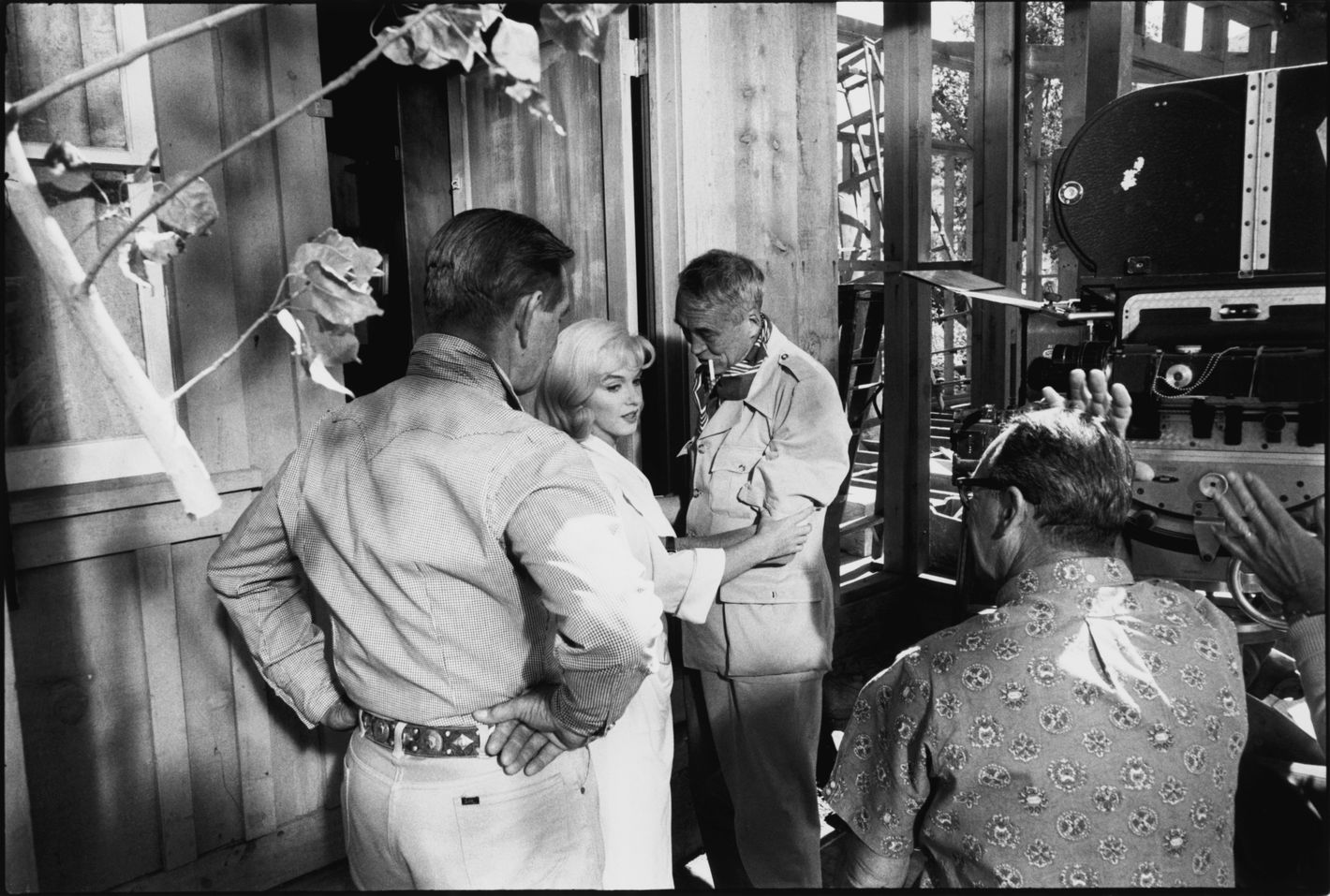This is a black and white image capturing a scene from a movie production, set in what appears to be a wooden barn or cabin. In the center of the shot, Marilyn Monroe, wearing a white collared shirt dress, is in a semi-embrace with an older man dressed in an old-timey suit. The man has a cigarette hanging from his mouth and is looking down at her, while she gazes towards the camera. To the right, a crew member wearing a floral short-sleeve shirt and glasses observes the scene. Another man, standing on the left with a studded belt and hands on his hips, looks on as well. The perspective of the image is from behind a large camera, with sunlight illuminating the backs of some crew members. In the background, branches and sunlight enhance the rustic feel of the setting.